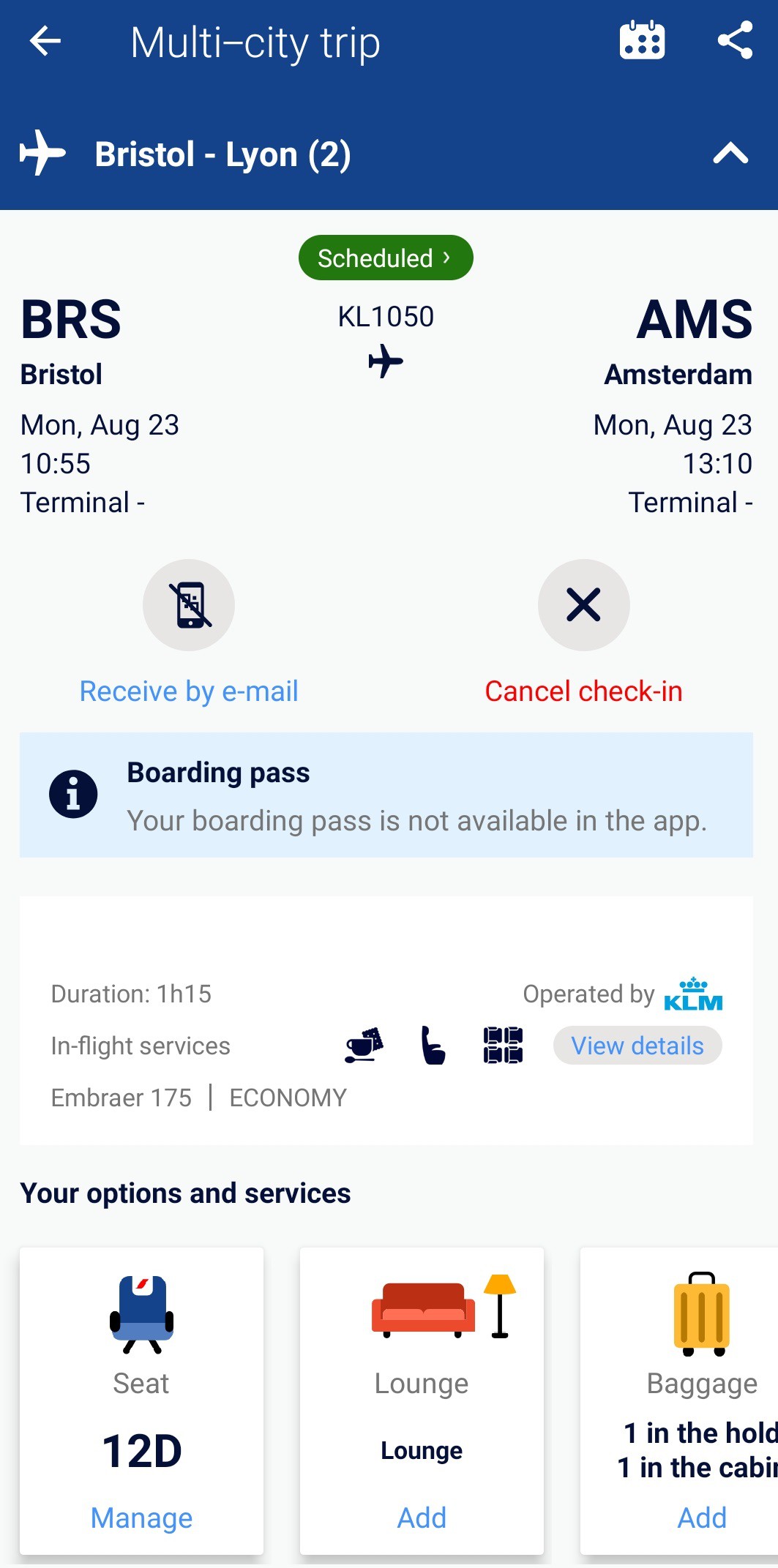This screenshot provides a detailed overview of a multi-city trip itinerary, displayed within a blue header. Adjacent to the header, there are icons representing a calendar and sharing options. Below this, an image of an airplane is displayed, along with the text "Bristol to Lyon (2)" and an upward-facing icon. 

The next section pertains to flight details, beginning with a flight from Bristol (BRS). The departure is scheduled for Monday, August 23rd at 10:55 AM, from the terminal, under flight number KL 1050, indicated by an airplane icon beneath the text. This flight heads to Amsterdam (AMS), arriving on Monday, August 23rd at 13:10 in the terminal.

Further below, two icons are shown: "Receive by Email" and "Cancel Check-in." A light blue rectangle labeled "Boarding Pass," accompanied by an information icon, states that the boarding pass is not available within the app. Beneath this, within a white rectangle, it specifies the flight duration as 1 hour and 15 minutes, along with the in-flight services. The text further indicates the aircraft type as Embraer 175 in economy class, operated by KLM, with a button to view additional details.

Several icons are also featured, including a teacup, an airplane seat, and what appears to be a parking icon. The section labeled "Options and Services" specifies seat 12D, offering a "Manage" option with an airplane seat icon. Additional options include "Lounge" featuring a red couch icon and "Baggage" which details "one in the hold and one in the cabin" illustrated by a small yellow suitcase.